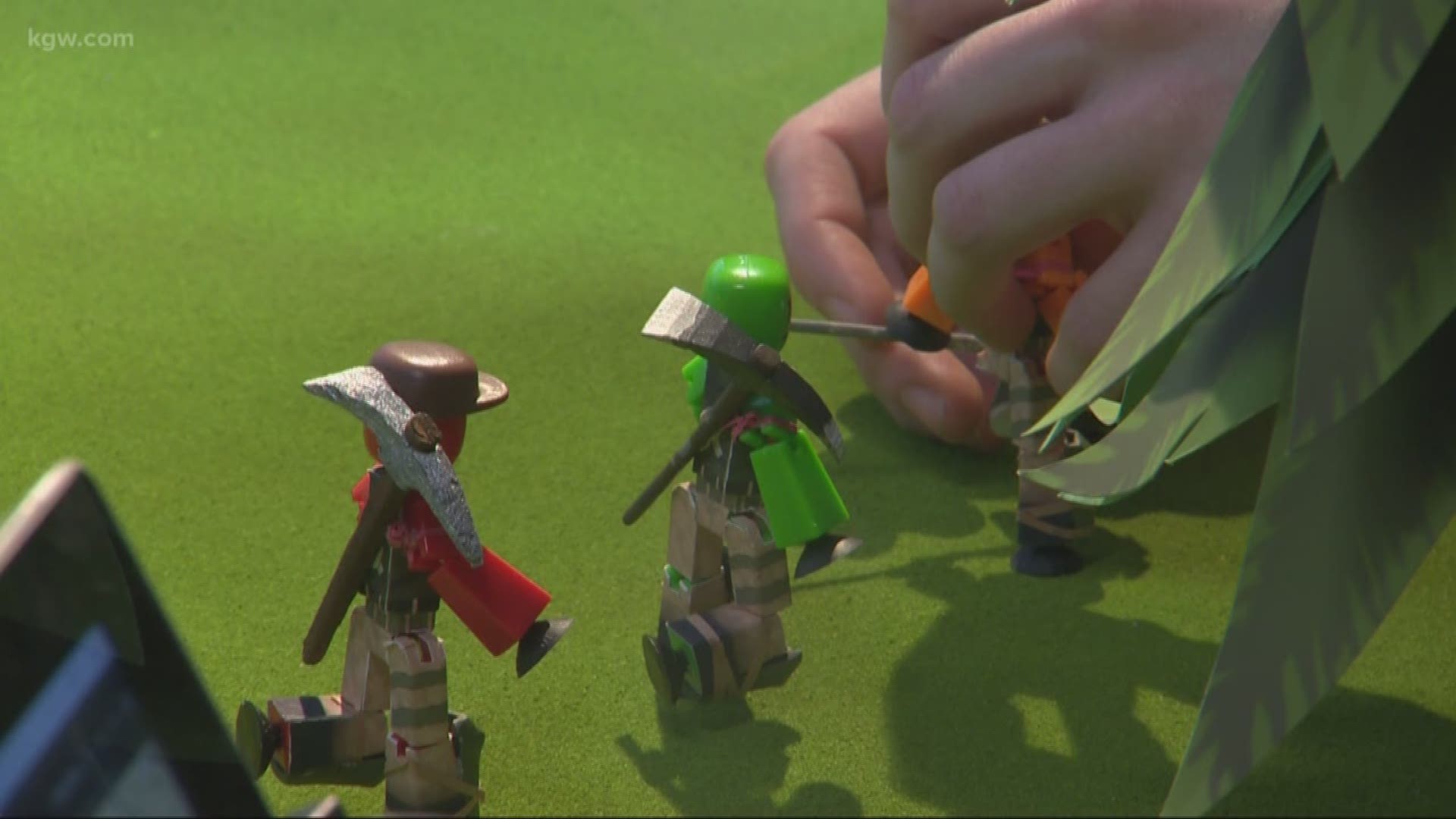This outdoor photograph captures a scene where someone is setting up a miniature play area on a green, felt-like surface, possibly for a stop-motion animation project. Three small, humanoid toy figures are prominently featured: the leftmost figure wears a red shirt with camouflage pants and a hat, carrying a makeshift pickaxe; the middle figure is clad in a green helmet and shirt, also with a pickaxe on its back; the rightmost figure is orange, partially obscured by a pair of hands adjusting it, and appears to have a wooden lower body. To the right of the scene are artificial green leaves resembling those of a pine or palm tree, and in the bottom left corner, a screen device, possibly a computer or iPad, displays the text "KGW.com." The figures appear to be in motion, either running or marching, set against a backdrop that enhances the meticulous and creative nature of the project.